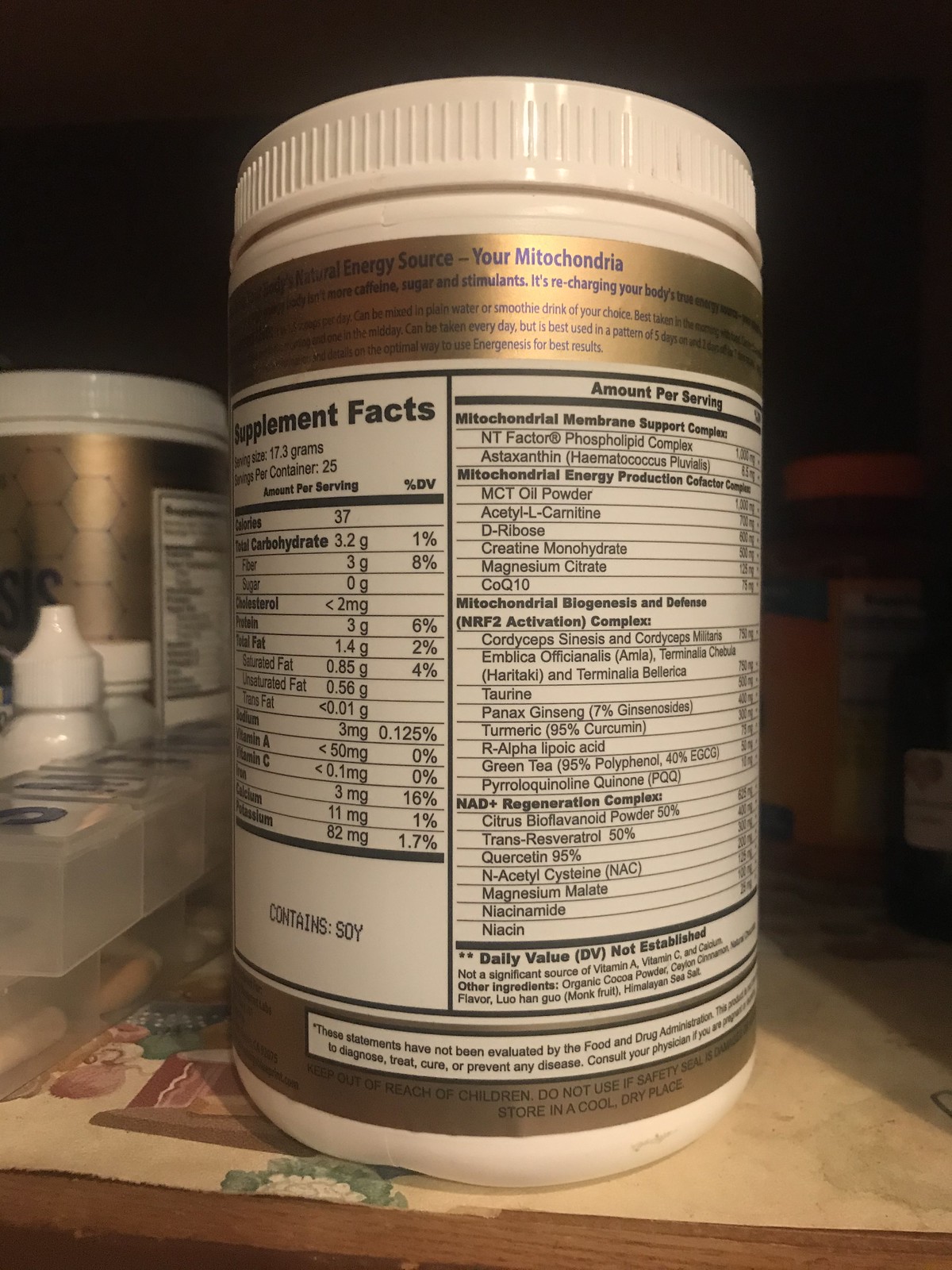Photograph of a plastic supplement bottle prominently displayed in the center. The bottle's label is facing backward, showing the 'Supplement Facts' section, although the text is largely blurry and illegible. To the left of the main bottle, there are several smaller containers, including what looks like a squeeze bottle, possibly for liquid drops. Another small supplement bottle appears to be partially obscured behind the squeeze bottle. Additionally, a small item resembling a pill dispenser is situated among the smaller bottles. The arrangement suggests a diverse collection of health-related products, though the specifics remain indistinct due to the blurriness of the image.